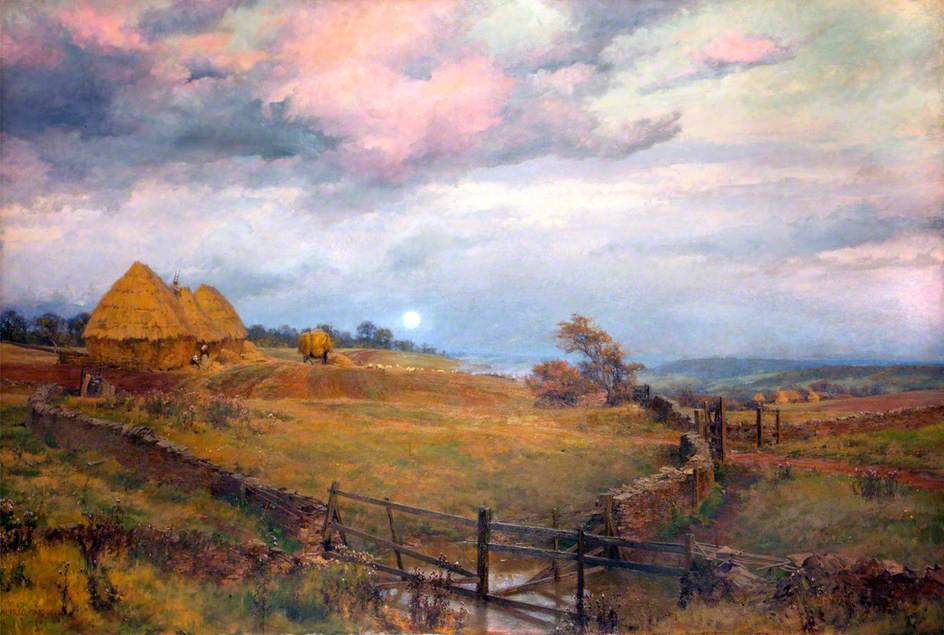This painting depicts a serene, rustic landscape showcasing a grassy meadow with long greenish-brown grass characteristic of late fall. To the left, three straw huts, possibly made of hay, stand on a slight elevation, with what appears to be a wagon nearby. The meadow is divided by a combination of stone and wooden fences, one of which leads to a small, somewhat broken wooden gate that opens into a tranquil creek or a large puddle. To the right, additional grass huts can be spotted lower in the scene. The landscape is composed of rolling hills that dip into a valley, suggesting higher ground on which the viewer stands, with a distant body of water or perhaps another valley. The horizon is lined with trees beneath a mostly cloudy sky, featuring colors that shift from soft pinks and golds to purples and blues, reflecting the setting sun. The sky's beauty is accentuated by thick, puffy clouds, creating a calm, picturesque backdrop as the moon subtly rises in the distance.